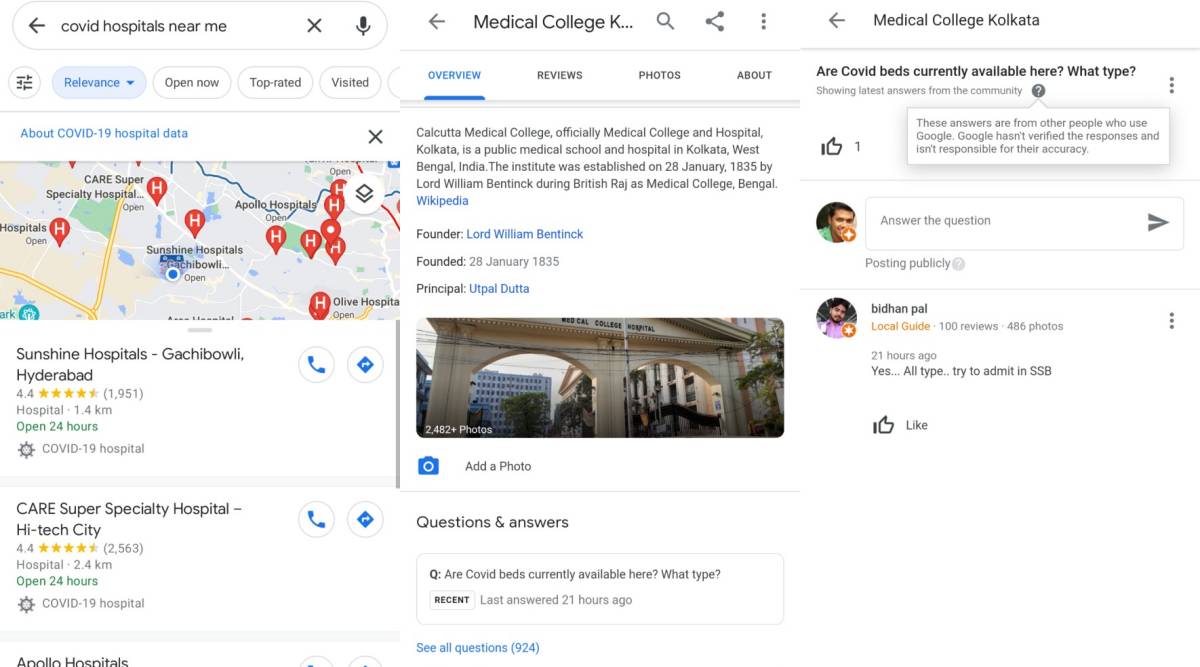This image is a composite of three screenshots, each providing information related to hospitals and medical colleges. 

1. The first screenshot captures a search query for "COVID hospitals near me." The visual includes a map marked with red location pins labeled with "H" icons, indicating hospital locations. Notable mentions are Sunshine Hospital in Gachibowli, Hyderabad, and Care Super Speciality Hospital in Hitech City.

2. The second screenshot showcases a snippet about "Medical College K," clarifying its full name as "Calcutta Medical College." The description, sourced from Wikipedia, details that it is officially known as Medical College and Hospital, Calcutta, a public medical institution in Kolkata, West Bengal, India. The college was founded on January 28, 1835, by Lord William Bentinck during the British Raj as Medical College, Bengal. The screenshot also features an image of the hospital entrance.

3. The third screenshot continues with a search query related to "Medical College, Kolkata," asking about the availability of COVID-19 beds. A response suggests that all types of beds are available, with a recommendation to admit at SSP. The response section includes two user icons, indicating it is part of a discussion or comment thread.

This comprehensive image amalgamation not only provides a quick overview of hospital options during the COVID-19 pandemic but also highlights historical and logistical details about key medical institutions.